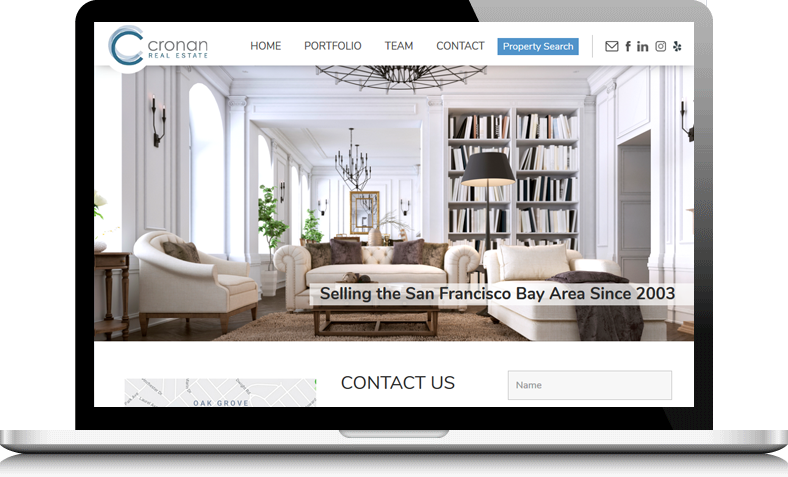The image is a detailed screenshot of a real estate webpage displayed on a laptop. The laptop, which has a black border and a slightly gray top right corner, is silver at the bottom and seen from a head-on angle with its screen open. The webpage has a white background with the title "Cronan Real Estate" at the top left, alongside a logo featuring three overlapping C's in varying shades of blue. Below this, a clean white menu bar lists options including Home, Portfolio, Team, and Contact, with a prominent blue button labeled Property Search.

The webpage also displays icons for popular social media platforms like Facebook, LinkedIn, Instagram, and Yelp. Dominating the screen is a large image of a luxurious, ornate living room. This room features plush white chairs and couches, exuding an air of opulence. The interior is predominantly white, complemented by two well-stocked bookshelves, a black lamp, and a brown rug. To the right, there's a doorway and elegant black chandeliers hanging in the background. The room is further adorned with indoor plants, adding a touch of greenery. In the bottom right corner of the image, a white text box states "Selling the San Francisco Bay Area since 2003." Below the main image, the page continues with a clean white background featuring “CONTACT US” prominently in black capital letters.